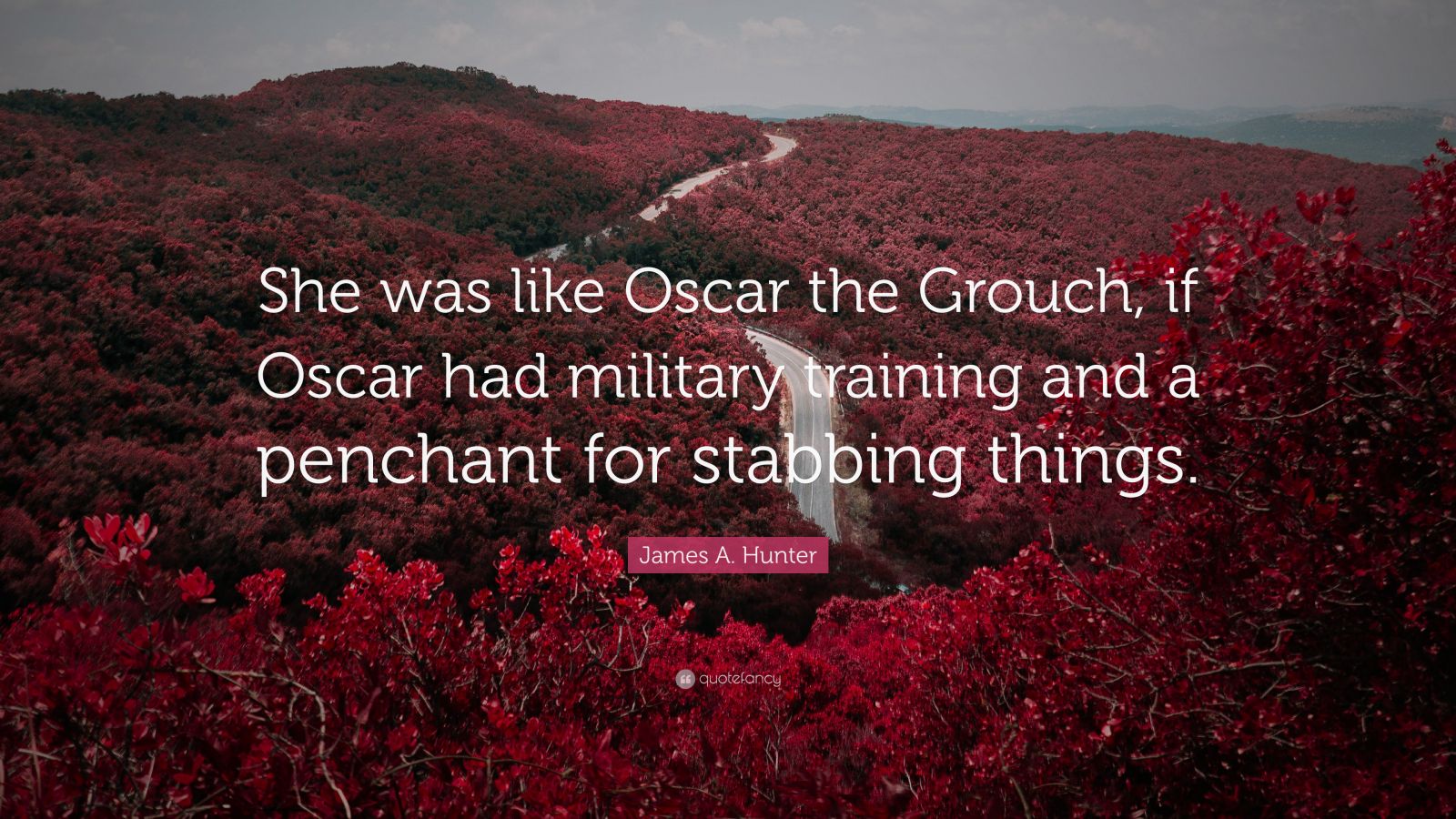The image features a dramatic natural landscape dominated by vibrant, crimson red foliage, resembling trees or bushes, which blanket a hillside or mountain. A river or road winds its way through the crimson landscape, adding depth and intrigue to the scene. The sky above is a moody gray, lending an air of melancholy to the setting. 

In the center of the image, written in large white text, is the quote: "She was like Oscar the Grouch if Oscar had military training and a penchant for stabbing things." Just beneath the quote, a red or deep pink rectangle contains the name "James A. Hunter" in white font. Below this, there is a circular watermark that reads "Quote Fancy" in somewhat hard-to-read gray lettering, accompanied by a quotation mark symbol. This overall scene feels typical of imagery often used for displaying profound or humorous quotes online.